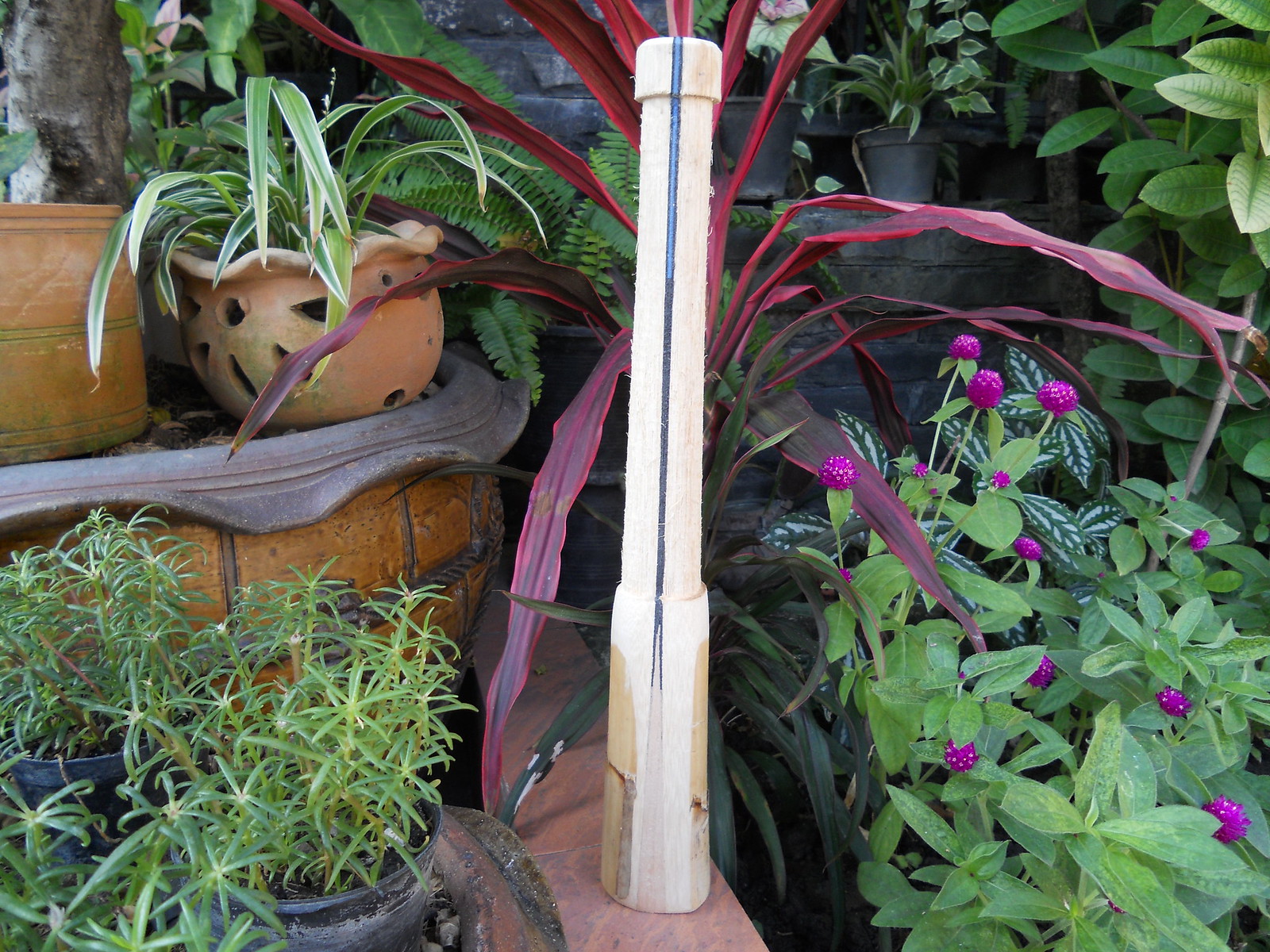This is an outdoor photograph of a charming, small garden area. Central to the image is a vertical, light-colored wooden post with a blue stripe, which visually divides the garden. In the top left, various plants are growing in orange, clay tile pots, one of which includes a jack-o'-lantern pot brimming with green vegetation. A smaller, empty orange pot sits nearby. In the bottom left, there are gray cauldron-shaped pots, containing shoots of grass and some weeds.

The right side of the garden features a spider plant with a pink hue, adding a touch of color alongside other foliage. There are also hosta plants with broad green leaves. A gathering of purple, dome-shaped flowers resembling echinacea adds vibrancy to the area. 

The background of the image includes a concrete or brick wall visible in the top right corner, framing the garden space. The garden as a whole has a serene, daytime ambiance, showcasing a mix of lush green plants and colorful flowers, all held within a variety of containers, creating a picturesque setting.